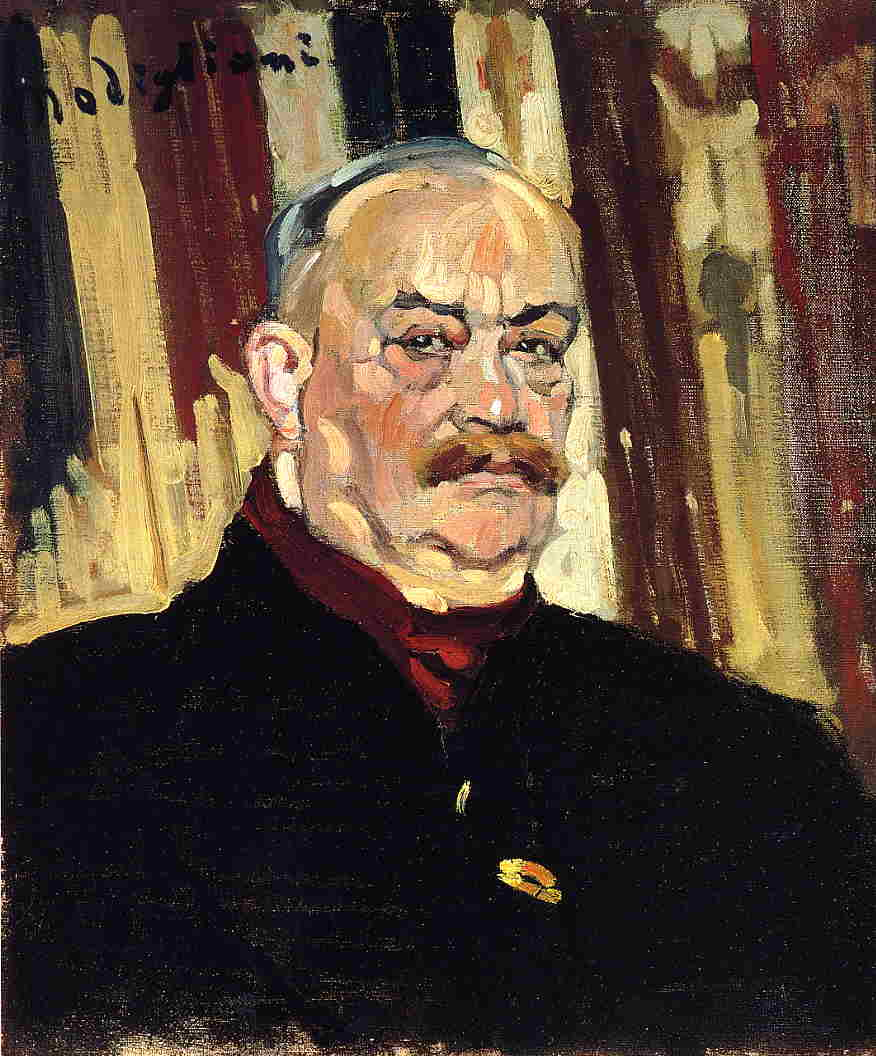This is a stern, middle-aged man depicted in a painting, with a receding hairline and thinning black hair towards the back of his head. He has intensely black eyebrows that are furrowed, piercing black eyes, and ruddy cheeks. His mustache is a distinct reddish-brown and parted in the middle, while his chin is also noticeably red. The man wears a dark overcoat over a burgundy shirt that extends up to his neck. Adding detail to his appearance, his neck is somewhat wrinkled, hinting at his age. He stands against a background of large, nearly vertical streaks of red, cream, and black, resembling the pipes of an organ. A signed name, likely "Modigliani," appears in the upper left corner of the painting. Overall, the man exudes a severe, intent expression as he faces the viewer directly.